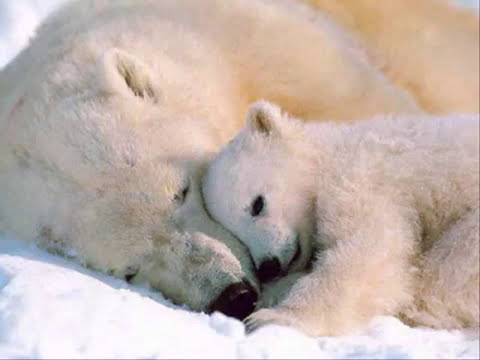In this close-up winter scene, a tender moment is captured between a polar bear mother and her cub nestled in the pristine snow. The adult bear, lying on her side with one ear peeking upwards, has a gentle tan tinge along her back, contrasting slightly against the stark white of their snowy habitat. Her cub, strikingly white and fluffy with expressive black eyes, nose, and mouth, rests its head lovingly on the mother's muzzle, one tiny paw reaching up towards her. The cub's eyes are half-open, suggesting gentle alertness while the mother appears to be in a sound sleep. Both bears display short, triangular ears with rounded tips, adding to their adorable appearance. The snow around them is pristine, whiter than their slightly dirty fur, which bears subtle eating stains, especially around their muzzles. A soft, reddish light casts a warm glow over their fur, emphasizing the snug, intimate setting of this serene winter wonderland.